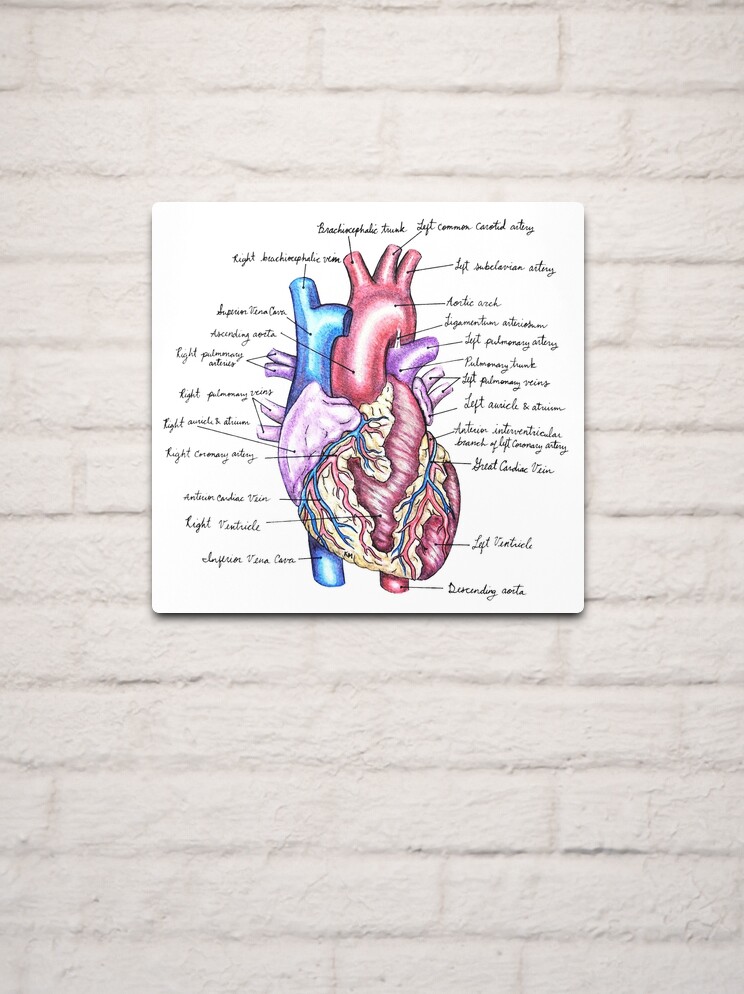The image features a detailed diagram of the human heart prominently displayed on a piece of white cardboard or canvas mounted on a white-painted brick wall. The heart is depicted with the left side in blue and the right in red, illustrating veins and arteries. Purple-colored structures represent the valves, while a pale yellow mass indicates fatty tissue near the bottom. The detailed anatomy includes labels in black script text pointing to various parts, such as the brachiocephalic trunk, left common carotid artery, left subclavian artery, aortic arch, left pulmonary artery, and more. The diagram appears as it might in an anatomy and physiology textbook, providing a clear and informative view of the heart's structure, including the great cardiac vein, descending aorta, interventricular branch of the left coronary artery, and the superior vena cava.